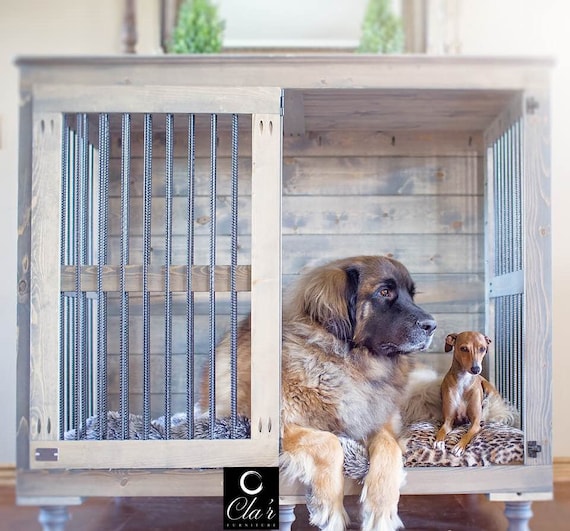This image showcases a sophisticated dog crate made from a combination of wood and metal. The crate, featuring vertical metal bars and wooden panels, sits on a wooden floor against a tan beige wall. The front door of the crate is open, revealing two resting dogs. Above the crate, a window adorned with a drawn white curtain and flanked by two plants can be seen. The larger dog, positioned on the left, has light to dark brown fur with black accents on its ears and muzzle, while the smaller dog on the right is primarily brown with a few white spots. Both dogs have their ears down and are lying on a cheetah-print cushion, gazing outside the crate. A logo reading "Shaz. C-L-A" in black with a white circle is visible at the bottom left, adding to the crate's luxurious design. The overall setting appears to be a cozy home interior.